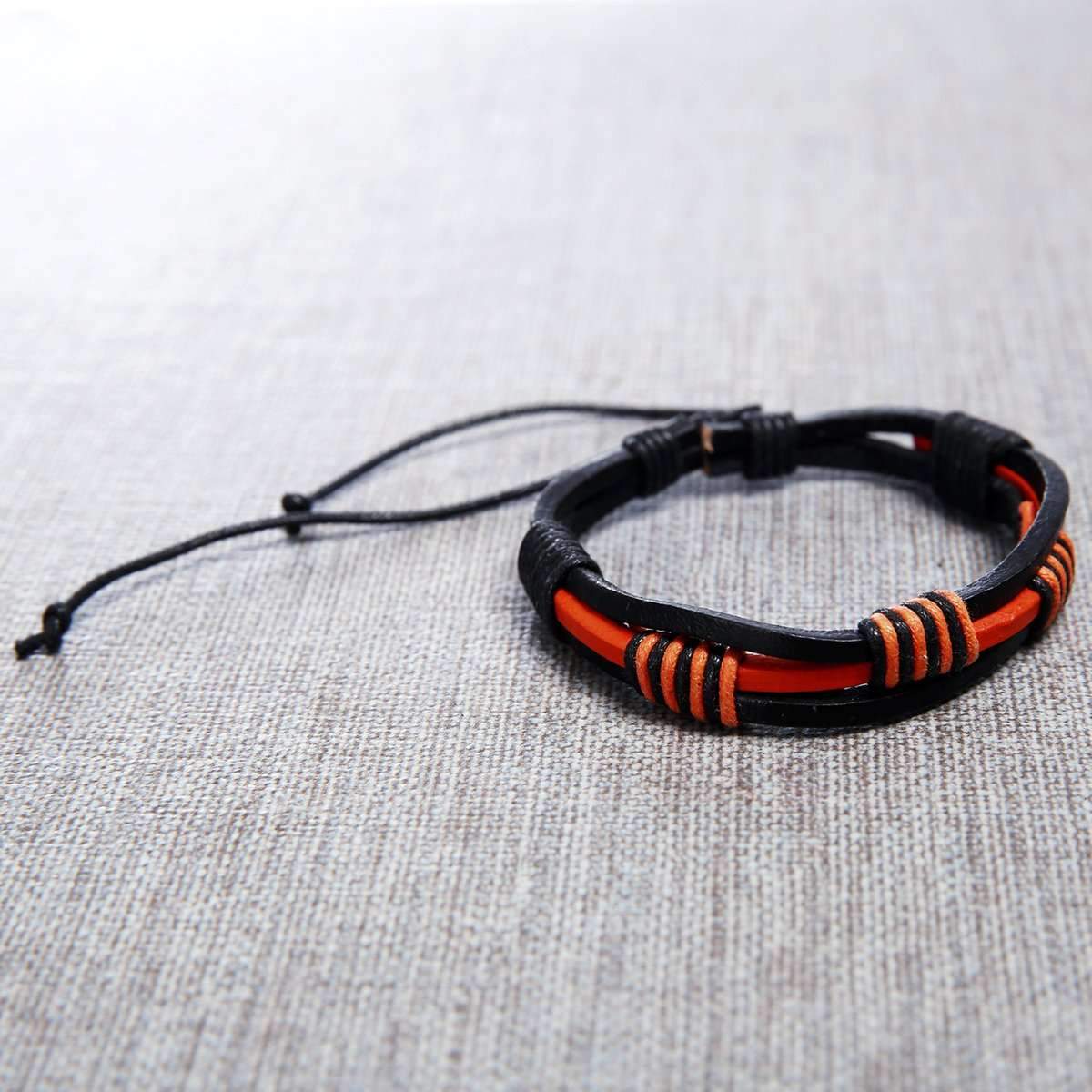The photograph showcases a handmade, adjustable leather bracelet prominently placed on the right side of the image. The bracelet rests on a grayish-white, short-fibered fabric, possibly linen or canvas. The bracelet is composed of three distinct layers of leather: a black layer on top, a red layer in the middle, and another black layer at the bottom. These layers are intricately connected by wrapped leather cords in a decorative pattern, featuring small bands of orange and black leather which give the bracelet an aesthetic reminiscent of red and black licorice. Two longer pieces of leather cord, ending in knots, trail off to the left side of the photograph. These cords, approximately four inches long, allow for the bracelet's adjustability. The black and red leather has a noticeable sheen, adding to its masculine appearance.